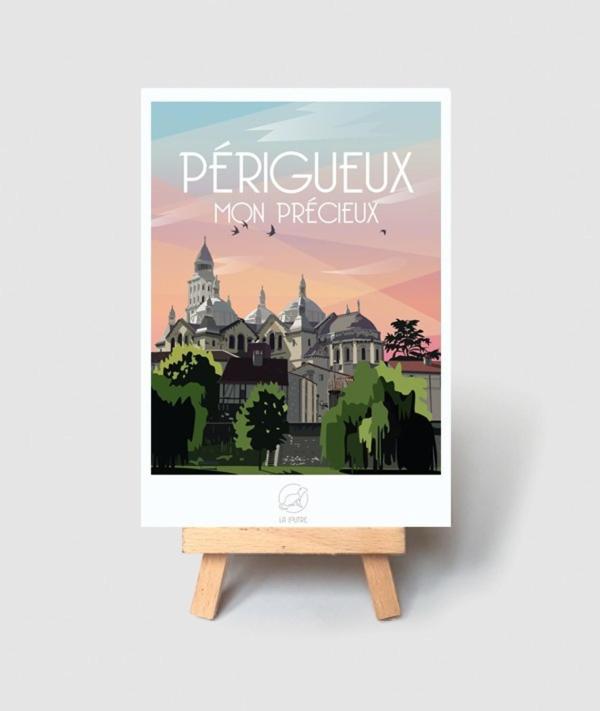This image features a light gray to whitish-gray background with a centrally positioned picture resembling a poster, framed by a white border thicker at the bottom. The poster is placed on a pine-colored wooden easel. The artwork on the poster is an abstract illustration of a large, castle-like building with numerous sections and several domes topped with points and steeples. The sky behind the building is a blend of blue and peach hues, adding to the artistic feel. Surrounding the base of the building, trees and greenery are depicted, particularly in the lower left and right corners, with a grassy patch at the bottom. There appears to be a French text, possibly "Périgueux, Mon Précieux," at the top in white. Additional text at the bottom, although illegible, further adds to the poster's detail. The entire setup suggests a hypothetical or artistic display rather than a real scene.